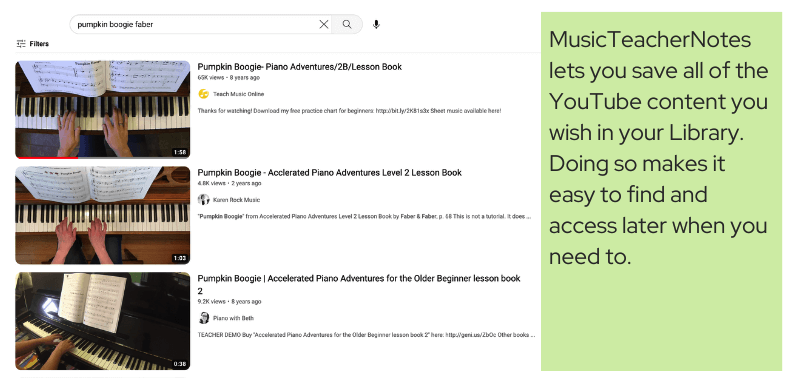The image features a search bar at the top with the query "Pumpkin Boogie Paper." Below the search bar, three YouTube video thumbnails are displayed. Each thumbnail showcases a piano with sheet music resting on it and a person's hands poised to play. The titles of the videos provide different instructional levels for the piece "Pumpkin Boogie": 

1. "Pumpkin Boogie Piano Adventures Level 2 Lesson Book"
2. "Pumpkin Boogie Accelerated Piano Adventures Level 2 Lesson Book"
3. "Pumpkin Boogie Accelerated Piano Adventures for the Older Beginner Lesson Book 2"

Beneath each video title, there is a brief description, the number of views, and the date it was posted. On the right side of the screen, there is a light green box with black text that reads: "Music Teacher Notes lets you save all of the YouTube content you wish in your library. Doing so makes it easy to find and access later when you need to." Next to the search bar, there is an 'X' icon and a magnifying glass icon.